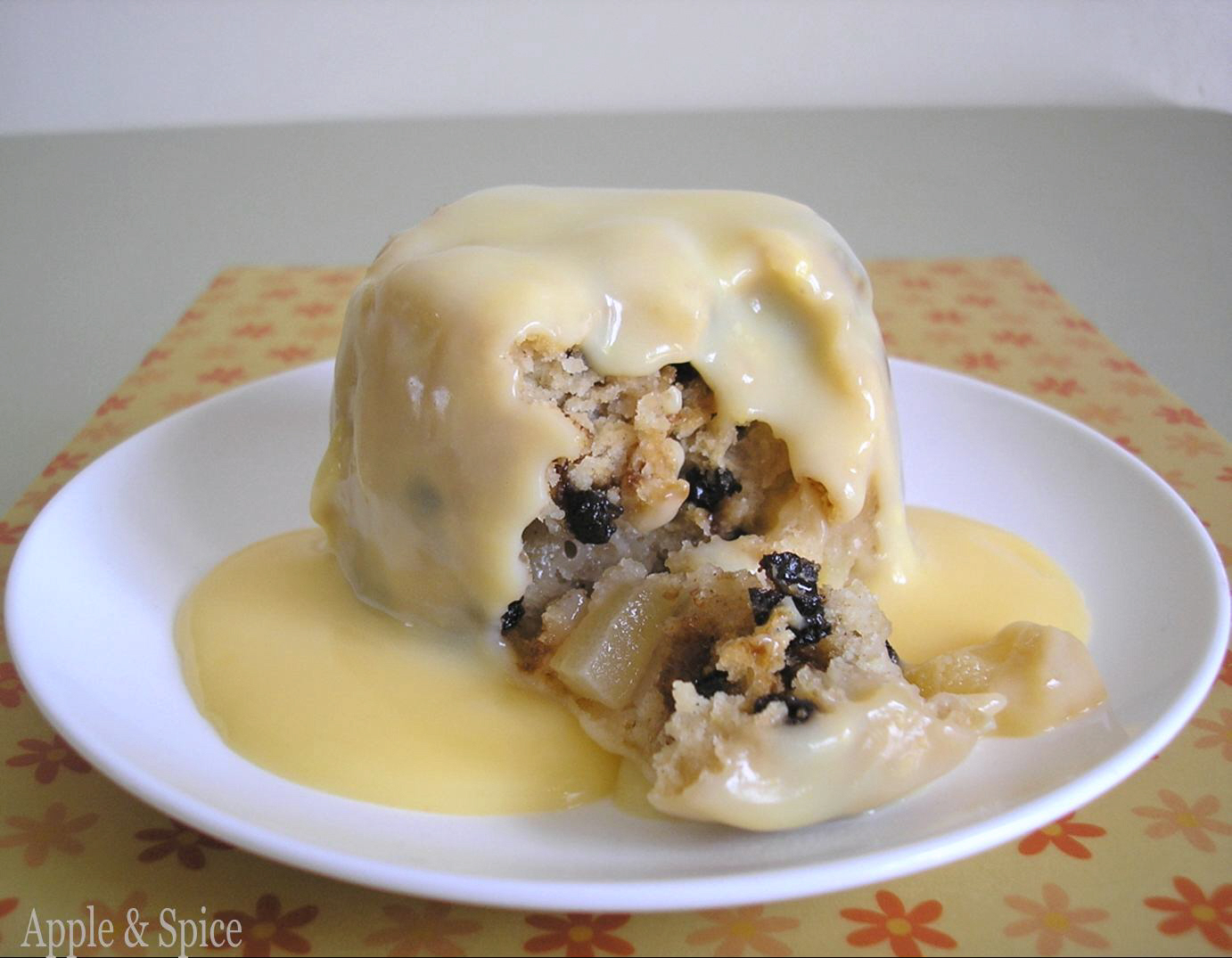The image showcases a gray table adorned with a vibrant placemat featuring a cream-colored background and a repeating pattern of six-petaled flowers in shades of orange and pink, each with a yellow center. At the center of the picture is a circular white plate displaying a piece of dessert, which appears to be an apple cake. The cake is generously covered in a creamy, gooey frosting that drips over the sides, forming a small pool on the plate. A piece has been cut open, revealing the interior texture, which includes chunks of apple, raisins, and possibly oatmeal or blueberries. The bottom left corner of the image has a label stating "apple and spice," indicating the flavor of the dessert. The overall scene presents a nostalgic, almost 70s-style aesthetic with its floral placemat and detailed food presentation.